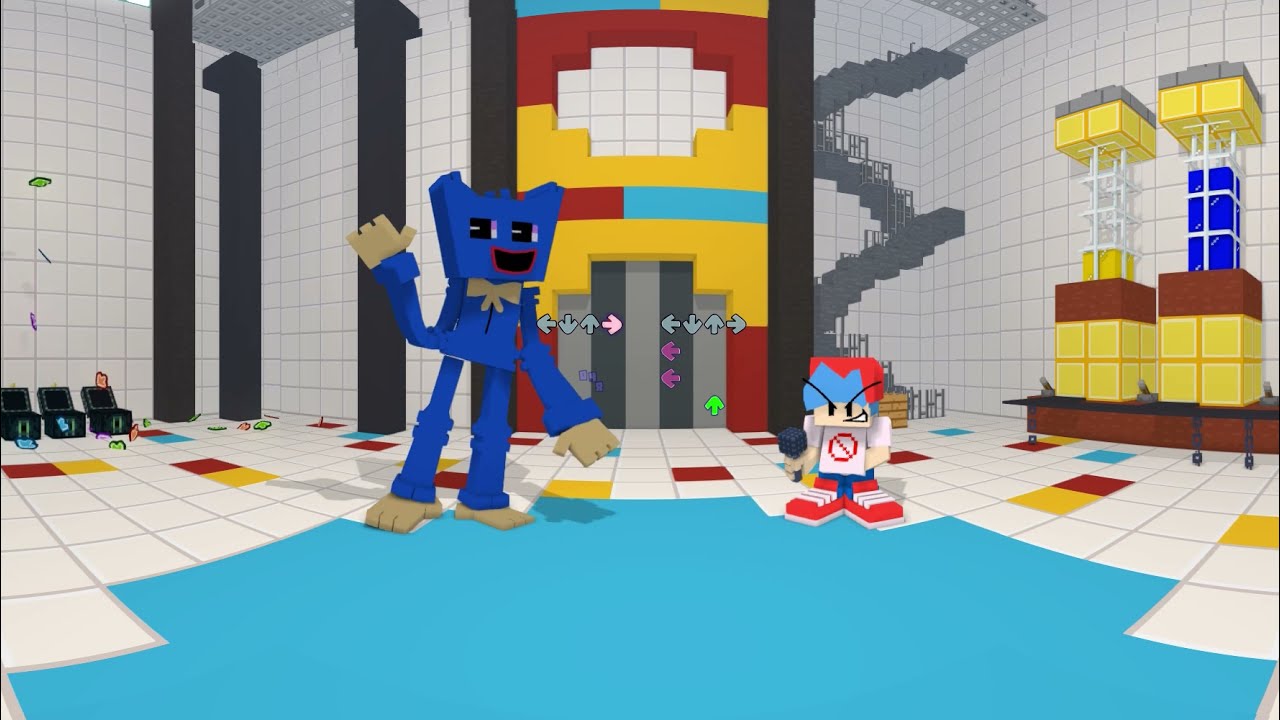This is a detailed screenshot from an animated video game, depicting a scene within a large tiled room. Two cartoonish characters stand at the center of the horizontally aligned rectangular image, on a multicolored tiled ground featuring light blue, white, yellow, red, and blue tiles. The walls of the room are made of white square tiles arranged in a gray grid pattern, with some black columns visible and a vibrant section above displaying yellow, white, and red colors.

On the left is a tall, blue, blocky character, distinguishable by its trapezoidal head, blue legs, blue arms, and gray feet and hands, also adorned with a gray bow tie. This character has small, black rectangular eyes with white dashes and a black mouth outlined in red. It appears to be waving with one hand.

To the right stands a smaller character dressed in a white shirt emblazoned with a red circle and a diagonal dotted line, complemented by blue pants and large red sneakers. The character has a blue head with red hair and tiny black eyes, and is holding a microphone.

In the background between the two characters is an elevator door, while on the left side, amidst some black chairs, there is a staircase leading upward. Notably, the scene is interactive, with arrows (up, left, side arrows) reminiscent of games like Guitar Hero, suggesting player interaction with the on-screen elements.